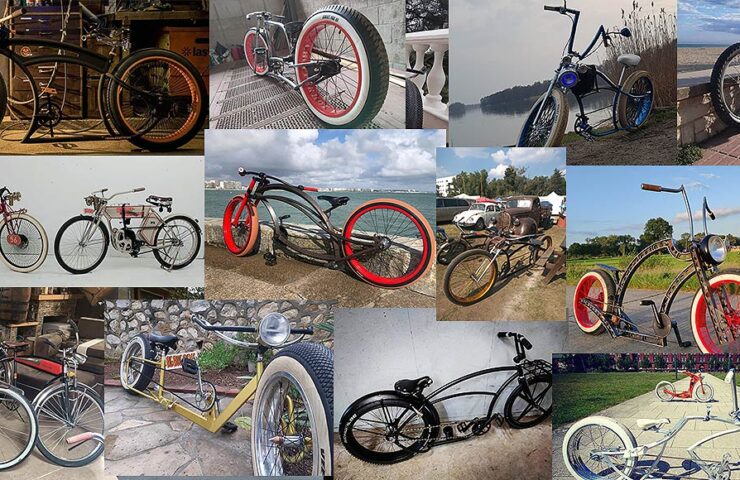This image is a collage of 12 bicycles, arranged in three rows of four pictures each. The pictures overlap, showcasing a variety of unique and traditional bicycles in different settings. In the upper left corner, there is a black bike missing its front wheel, resting in a garage. Next to it, there's a long bike with a thick rear wheel featuring a red and white rim. Another bike in this row has long handlebars, handbrakes, and gray, thick wheels. The rightmost image in the top row displays part of a wheel with a body of water in the background.

The middle row continues with a diverse selection: a white bike, an orange bike, and a brown one can be seen, as well as an eccentric bike with a highly curved frame and extended handlebars. There's also an image of a bike with a red frame and matching red wheels, black handlebars with red tips, and a black seat with an elongated area between the seat and handlebars. This bike has a unique bent frame to accommodate its length.

The bottom row features more distinctive bicycles. Among them is a futuristic-looking bike with a white seat and blue light in the front. Another bike in this row has red interior tires and a white-walled design, set against a grassy field. There's also a standard road bike with fenders and a front carrier, and lastly, two unconventional bikes that stand out for their atypical designs.

Overall, this collage exhibits a mix of indoor and outdoor settings, highlighting the diverse styles, frame structures, and wheel sizes of the bicycles, ranging from traditional to highly innovative designs.